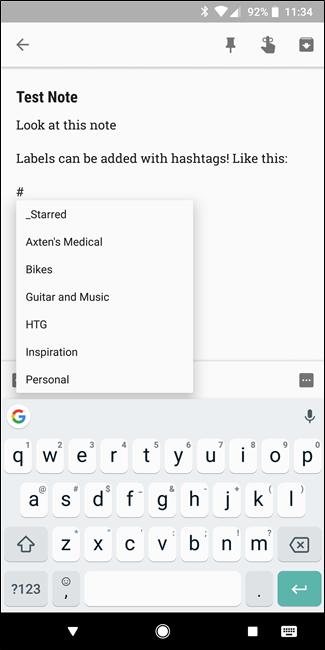This image is a screenshot taken from a cellphone. At the top of the screen, there's a gray status bar displaying various icons. On the right side of the status bar, the time is shown as 11:34, the battery is at 92%, and icons for Wi-Fi, cellular signal, and Bluetooth are visible. The left side of the status bar is empty except for the gray background.

Below the status bar, there is a navigation arrow pointing left, followed by a pin icon, and a reminder symbol represented by a finger with a ribbon around it. Below these icons, a note is displayed within a text box. The note reads: "Test Note. Look at this note. Labels can be added with hashtags like this." A hashtag symbol (resembling a tic-tac-toe board) is also present.

A pop-up box under the note lists various labels, such as: "_starred," "Axton's Medical," "Bikes," "Guitar and Music," "HTG," "Inspiration," and "Personal."

Towards the bottom of the screen, there's a Google search bar with the multicolored Google "G" icon on the left and a microphone icon on the right. Below the search bar is the mobile keyboard, featuring standard QWERTY layout keys, a space bar, a "123" key to switch to numeric input, a backspace key, and a row for navigation buttons at the very bottom. This row includes a triangle, a circle, and a square, each corresponding to different navigation functions. The bottom area of the screen is black, providing a contrast to the keyboard and icons.